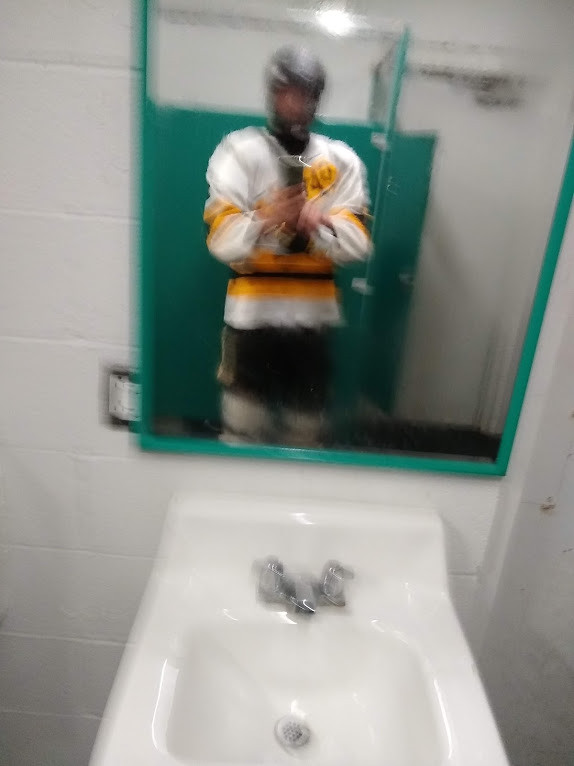In this blurry photograph, a man is taking a selfie in the mirror of a bathroom. The background consists of a white painted cinder block wall. Central to the image, at the bottom, is a white porcelain sink equipped with silver faucets. Above the sink, there is a rectangular mirror outlined in green. The reflection reveals the man holding his cell phone, standing against the gray metal walls of a bathroom stall.

He is wearing a black helmet and a white sports jersey featuring yellow and black lines. His attire is completed with black shorts, and though it's difficult to discern, there appears to be something white on his thighs. Above his head, in the mirror's reflection, a round, bright light is prominently visible, adding to the overall illumination of the scene.